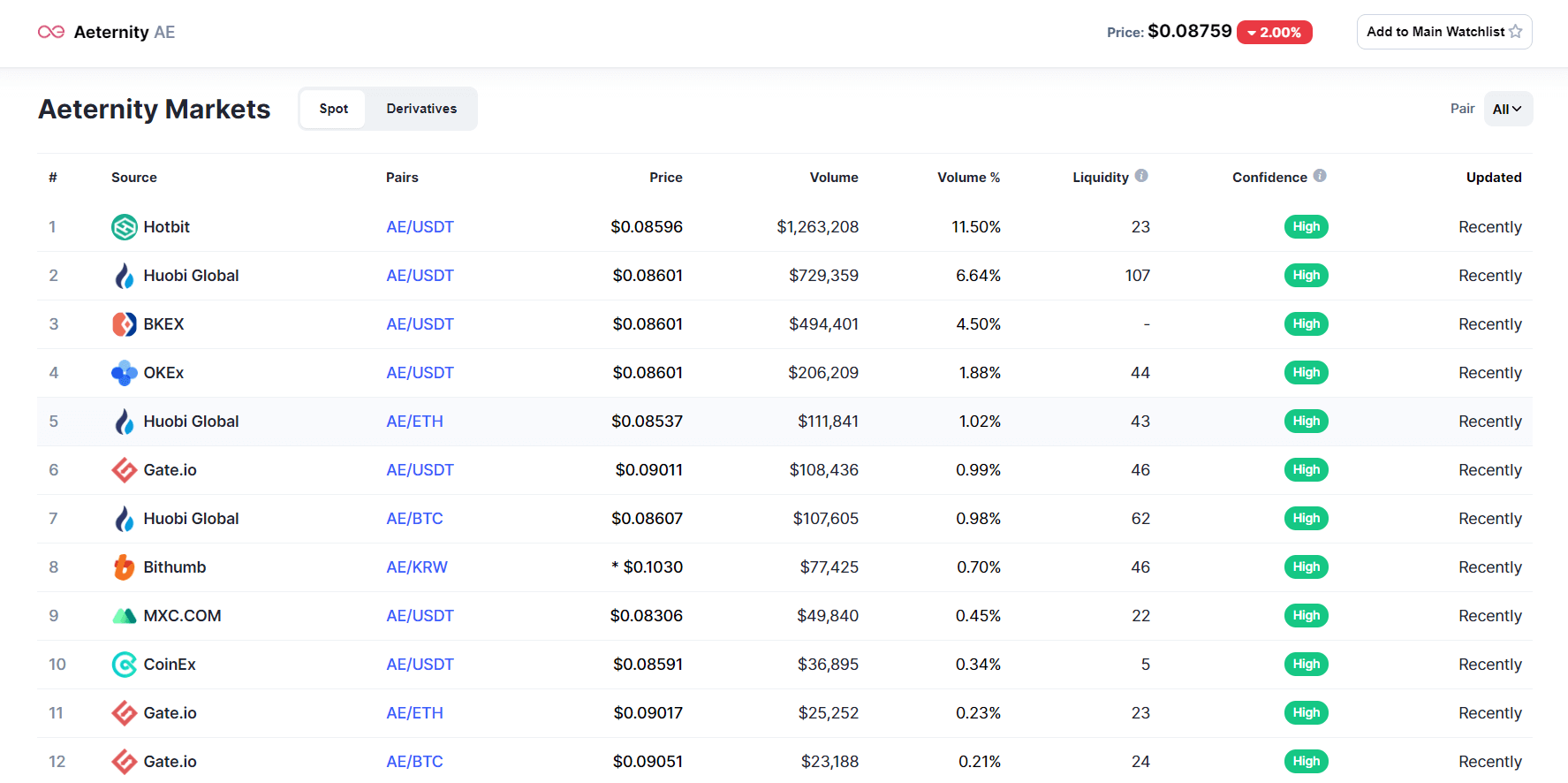In this image titled "Aeternity," we see detailed information about the cryptocurrency displayed prominently. The name "Aeternity" is positioned at the top left corner of the image, spelled out as A-E-T-E-R-N-I-T-Y. The name is highlighted on a white bar that stretches horizontally across the image. On the right end of this white bar, the current price of the cryptocurrency is listed as 0.08759. Just beside the price, there is a downward-facing red arrow accompanied by a percentage figure indicating a 2.00% decrease. To the right of this is an option to add Aeternity to the main watch list.

Below the white bar is a section titled "Aeternity Markets," which contains a detailed table of 12 different market sources for this cryptocurrency. Each row in this table lists the following columns: Source, Pairs, Price, Volume, Volume Percentage, Liquidity, Confidence, and Last Update. The first entry in this table is from the source "Hotbit," showing a price of 0.08596 and a trading volume of $1,263,208. The entire image provides a comprehensive snapshot of the current state of Aeternity in various markets.